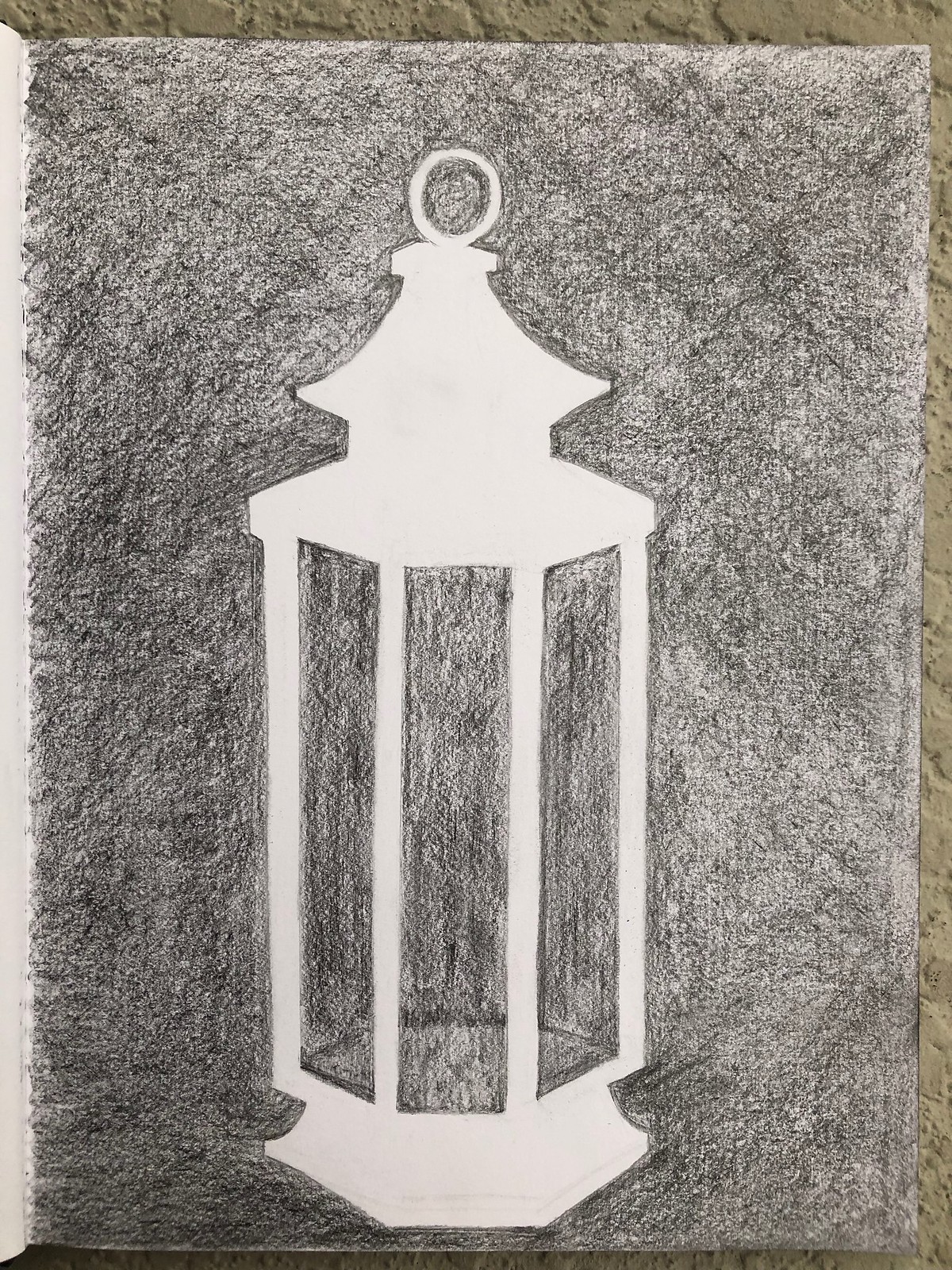This charcoal drawing features a detailed depiction of a lantern rendered in a distinctive inverted style. At the top of the lantern, a circular hook adds a functional touch, complemented by a curved, flared upper section that transitions into a more angular, squared-off portion. Below, a hexagonal shape forms the upper part of the lantern, with four definitive lines extending downwards, representing the structural supports that would typically house glass panels. The base of the lantern features an elegantly curved, outward-angled design, leading into another multi-angled segment at the bottom. What makes this artwork particularly intriguing is the technique used: the artist has filled the entire paper with a pencil charcoal shading, leaving the lantern itself untouched in white. This negative space approach creates a striking contrast, making the lantern stand out vividly against its dark background.